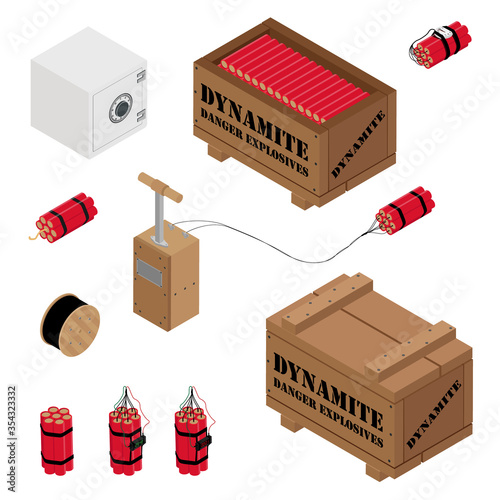The image is a detailed computer-generated rendering showcasing various elements related to dynamite, all set against a white background. Featured prominently is a white safe in the upper left corner. Adjacent to the safe, there's an open wooden box labeled "Dynamite" with a warning text that reads "Danger Explosives." Inside and around the box are several sticks of red dynamite. To the right of the open box is a bundle of dynamite sticks already connected with wires. Below this setup, another similar bundle of dynamite is attached by wires to a wooden platform equipped with a lever, designed to trigger an explosion. Additionally, there are several more dynamite sticks bundled with black tape into groups of seven. Scattered throughout the image, these elements are organized yet not centrally aligned, suggesting a meticulous yet somewhat chaotic arrangement. The colors dominating the scene are brown, red, white, silver, gray, and black. This detailed arrangement, including both open and closed boxes of dynamite, along with various wired components, suggests the image could be purposed for educational or illustrative use, possibly for a site concerning explosive ordnance.